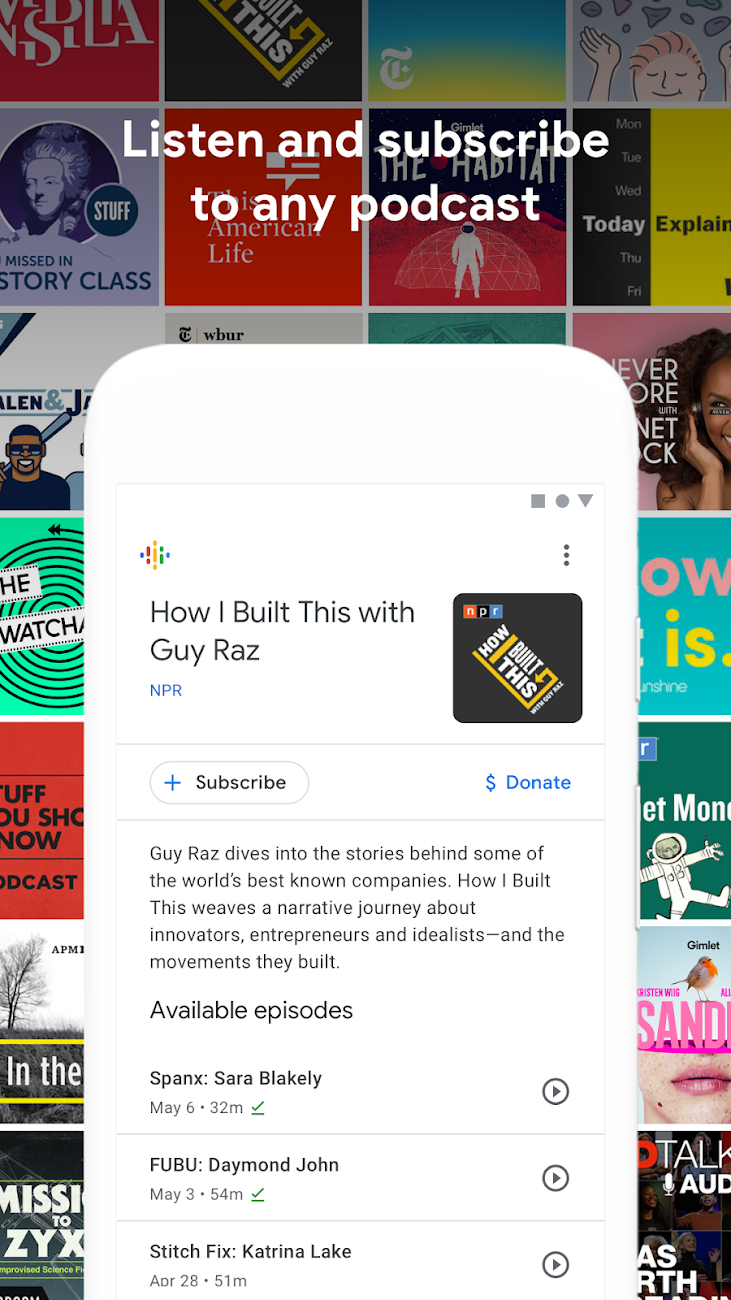The image features a diverse array of colorful, square-shaped boxes spanning from left to right at the top part of the composition. Each box contains different colors and elements within them, for instance, a red box is positioned at the top, adjacent to a light purple box on the left and a black and red box on the right. Further to the right lies a yellow and black box. These medium-sized boxes are neatly aligned next to each other, showcasing various texts, shapes, and people.

Overlapping the red box at the top, there is white text that reads, "Listen and subscribe to any podcast." 

In the center stretching towards the bottom of the image, there is a prominent white vertical rectangular shape with rounded edges, resembling a smartphone. The outer part of this shape is white, and so is the screen, indicating that the phone is on. At the top part of the screen, black text states, "How I Built This with Guy Raz." To the right of this title, there's a rounded square box with white and yellow text in the center.

Beneath the title, a white oval button outlined in gray houses the black text "Subscribe." Continuing downward, black text provides a description: "Guy Raz dives into the stories behind some of the world's best-known companies. How I Built This weaves a narrative journey about innovators, entrepreneurs, and idealists, and the movements they build." 

Further below, a bolded heading in black text reads, "Available episodes." There are three rows listed under this heading:
1. Bank, Sarah Blakely
2. FUBU, Daymond John
3. Stitch Fix, Katrina Lake

To the right of each row, there are white circles outlined in gray with a gray arrow pointing to the right, indicating navigation options.